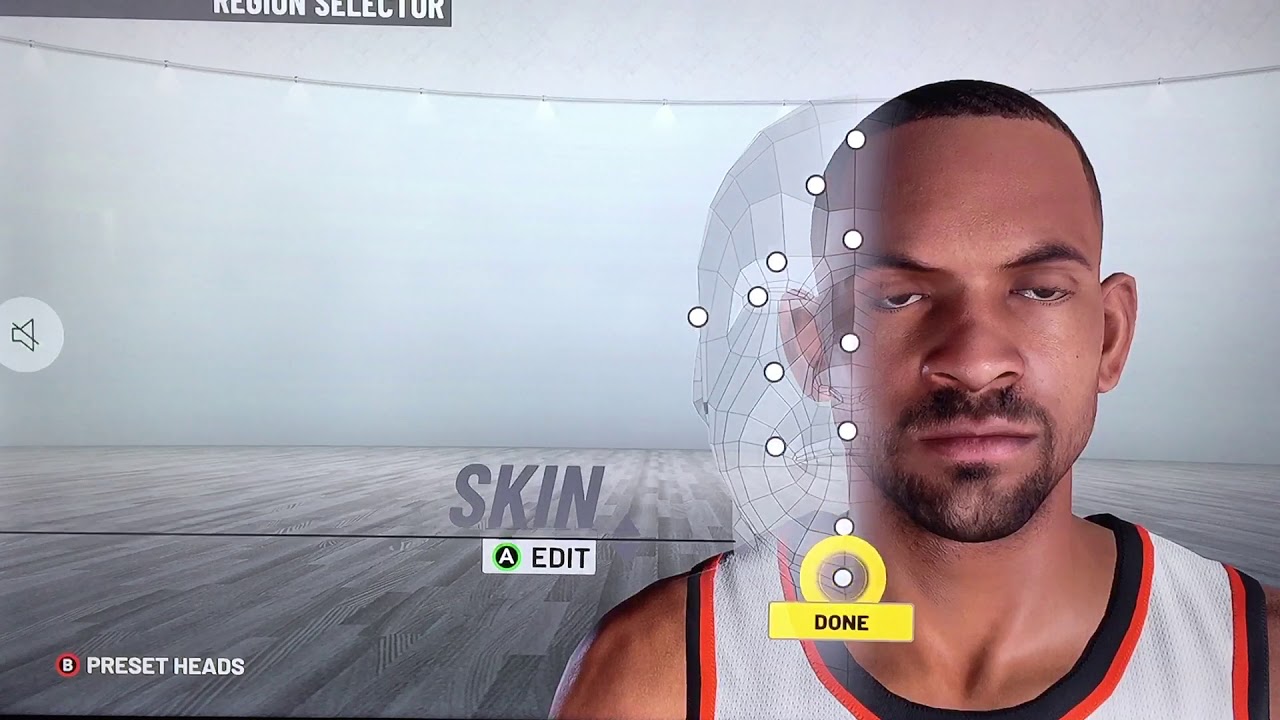This image captures a screenshot of a character editing interface, devoid of both header and footer. Dominating the right side of the frame is a highly realistic drawing, not an actual photograph, of a black man with medium brown skin. His hairstyle is characterized by very short black hair, complemented by a neatly trimmed beard and mustache. The man is clad in a light gray jersey, distinguished by orange and black trim.

Situated within the context of the editing page, the background is predominantly gray. Approximately two-thirds down the right side, behind the figure, the image intimates the portrayal of a gray floor. Overlaying the gray background, the term "SKIN" is conspicuously displayed in gray font. Directly beneath this text is a slightly off-white rectangle bearing the label "EDIT" in black font. Adjacent to this lies a gray circle outlined in a faint green hue, enclosing the letter "A."

Further to the right, various graphic overlays are discernible, including white dots and faint gray line renderings, reinforcing the interface's edit functionality. Towards the bottom, two prominent yellow shapes emerge: a circle and a rectangle, the latter inscribed with the word "DONE" in black font. In the lower-left corner, the phrase "PRESET HEADS" appears in white font. To the left of this phrase, an encircled letter "B" features a red outline, and to the right, a yellow circle is similarly encircled in red.